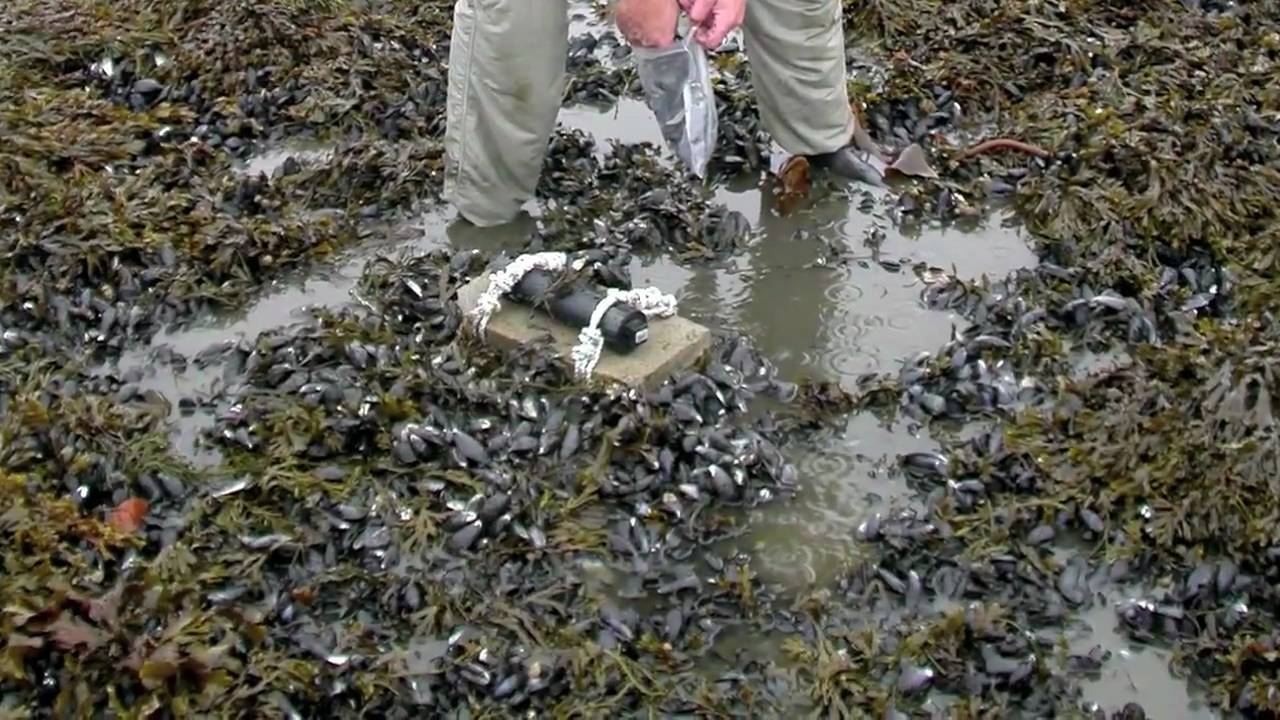The image depicts a marshy or swamp area, possibly during low tide or after a recent flooding. Within the murky, waterlogged environment that's dotted with patches of green moss and seaweed, we see a variety of black, elongated objects resembling seashells or mollusks with white-tipped ends scattered around. In the center of the image, there is a square gray stone block with a black cylindrical object strapped to it by white ropes. Standing in the ankle-deep water, a person wearing black boots, gray pants, and pink gloves is visible from the waist down. They are holding a silver and clear bag, into which they appear to be collecting something. The overall scene suggests an activity related to marine biology or shellfish harvesting.